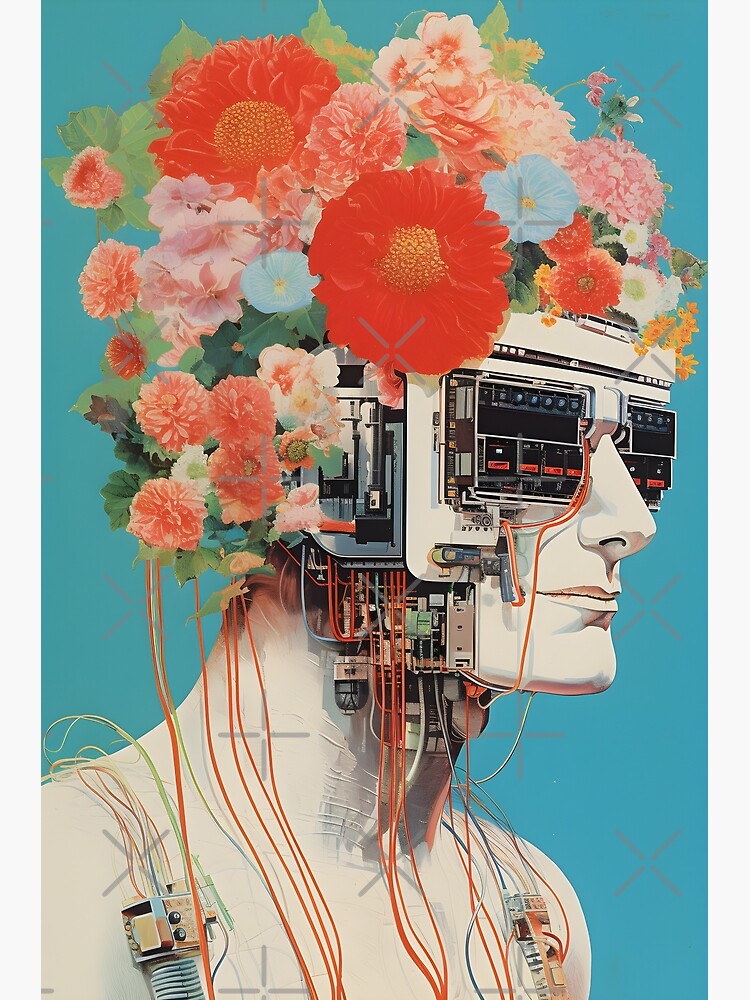This abstract art piece, likely created digitally, features a striking image against a light blue background framed by grey borders on the left and right sides. It portrays a hyper-realistic, mannequin-like face and upper body viewed from the chest or shoulders upwards, rendered in a metallic white or silver hue. The subject's head is adorned with a vibrant bouquet of orange, blue, pink, and white flowers intertwined with green leaves, substituting for hair. Additional detail includes small vines or wires hanging from the floral arrangement. 

The face reveals a stunning juxtaposition between organic and mechanical elements. The eyes are composed of intricate electronic components, including tape tracks, switches, buttons, and dials, resembling the interior of a computer tower. The right side profile showcases the nose and mouth as distinctly human features, while the ears and jawline incorporate circuit boards and wiring extending across the torso. Near the shoulders, the presence of additional electronic devices further blurs the line between the natural and the technological in this visually compelling and evocative piece of abstract art.